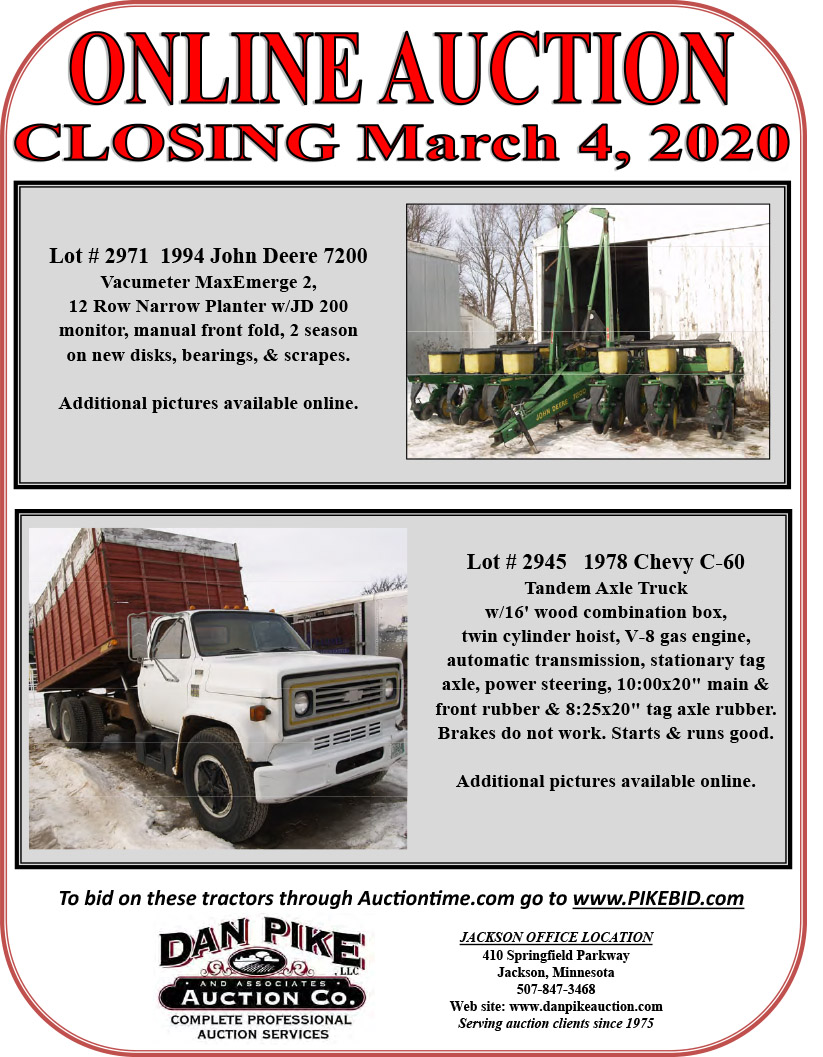This image is an advertisement for an online auction held by Dan Pike and Associates Auction Company, located in Jackson, Minnesota. The auction is closing on March 4th, 2020. Prominently featured are two main items: 

At the top, Lot number 2971 is a 1994 John Deere 7200 Vacu-Meter Max Emerge II 12-row narrow planter. This equipment includes a JD 200 monitor, manual front folds, and has two seasons on new discs, bearings, and scrapers. Additional pictures are available online. 

Below, Lot number 2945 is a 1978 Chevy C60 tandem axle truck. It has a 16-foot wood combination box, twin-cylinder hoist, V8 gas engine, automatic transmission, stationary tag axle, and power steering. The front rubber measures 10.00 by 20 inches, the tag axle rubber is 8.25 by 20 inches, and while the brakes do not work, the truck starts and runs well. Additional pictures of this item are also available online. 

For more details and bidding, visit www.danpikeauction.com or www.pikebig.com. Dan Pike Auction Company offers complete professional auction services out of their Jackson office located at 410 Springfield Parkway, Jackson, Minnesota, with the contact number 507-847-3468. The company has been serving auction clients since 1975, as illustrated by their logo displayed on the advertisement.